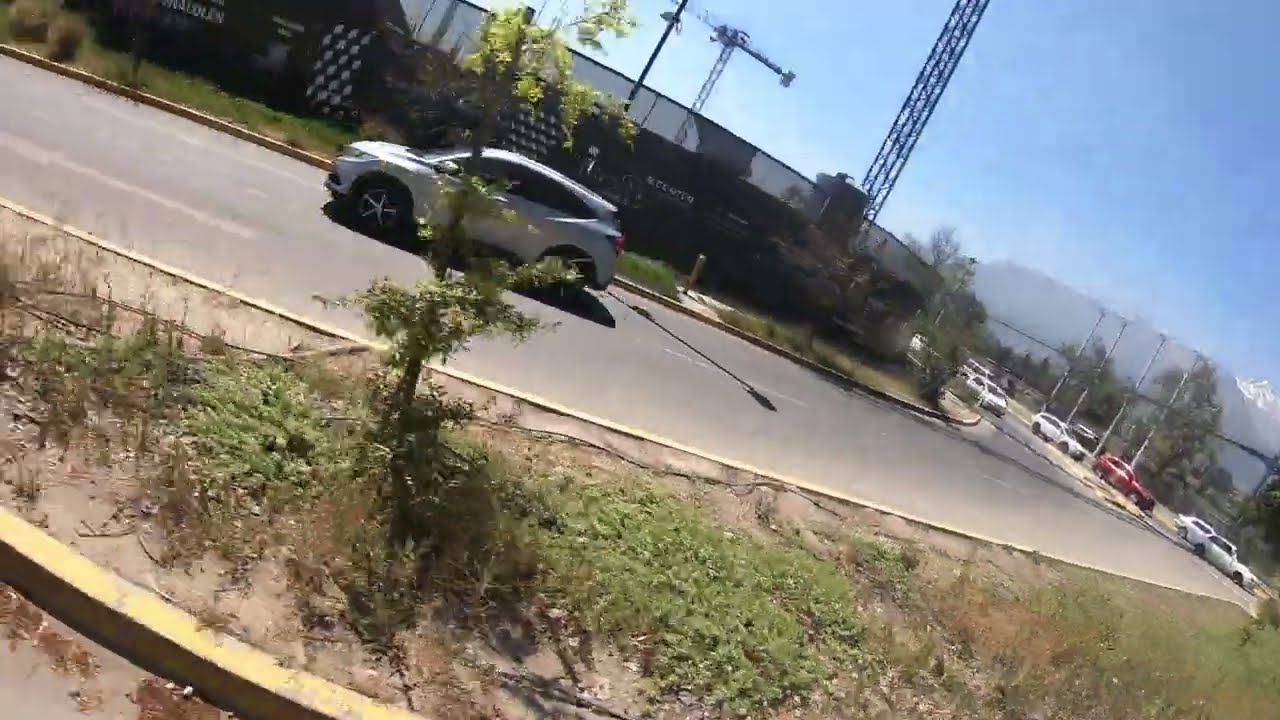The photograph captures a wide, rectangular outdoor setting focusing on a slanted road that stretches diagonally from the top left corner to the bottom right corner of the image. A silver SUV, capable of seating four people and sporting black tires with red tail lights, is prominently driving along this gray, paved street marked with white lines. The street is bordered by patches of unkempt land with dirt, sparse grassy areas, and small green trees, one of which appears to be falling apart. 

Adjacent to the road, a variety of cars, mostly white with a notable red one, are parked or arriving at what seems to be a construction zone or sports field, indicated by a dark, tall fence and visible cranes in the distance. Further back, another tall privacy fence encloses the area, adding to the sense of a restricted or private location. The background features a picturesque blue sky with a mountain range peeking through, adding a serene yet dynamic element to the otherwise ordinary scene.